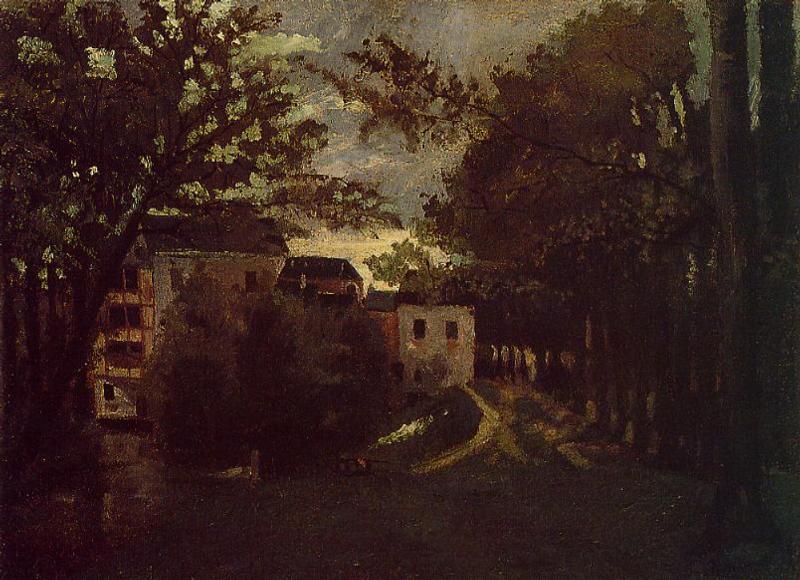This image is an oil painting depicting a somber, dusk-lit outdoor scene. The setting takes place at sunset, characterized by the rich oranges of the sun contrasting against the darkening blue clouds in the background. Silhouettes of tree branches and leaves frame the scene, adding depth and texture. Central to the painting is a two-story gray house with a black, sloping roof, accompanied by a nearby structure with a gabled roof. Adjacent to these is a taller, four-story gray building, also capped with a black roof.

The foreground is very dark, with indistinct shapes of trees bearing brown trunks and topped with a mix of yellow-green foliage and some barren branches, highlighted by bright green accents on a tree to the left. The right side features a grassy lawn leading to a small hill and a cluster of pine trees, while bushier yellow-green trees populate the skyline. A road or walkway meanders toward the central house, contributing to the serene yet slightly eerie ambiance.

Although the sky remains a focal point with its mixed hues of brown, umber, and dark grays achieved through wild brushstrokes, other details show a richly textured scene with numerous trees. These trees range from pine to leafy varieties, lining up on either side, while scattered houses in white and distant redbrick occupy the area behind clusters of foliage. The painting style strikes a balance between finely rendered details and impressionistic elements, giving it a unique and evocative atmosphere.